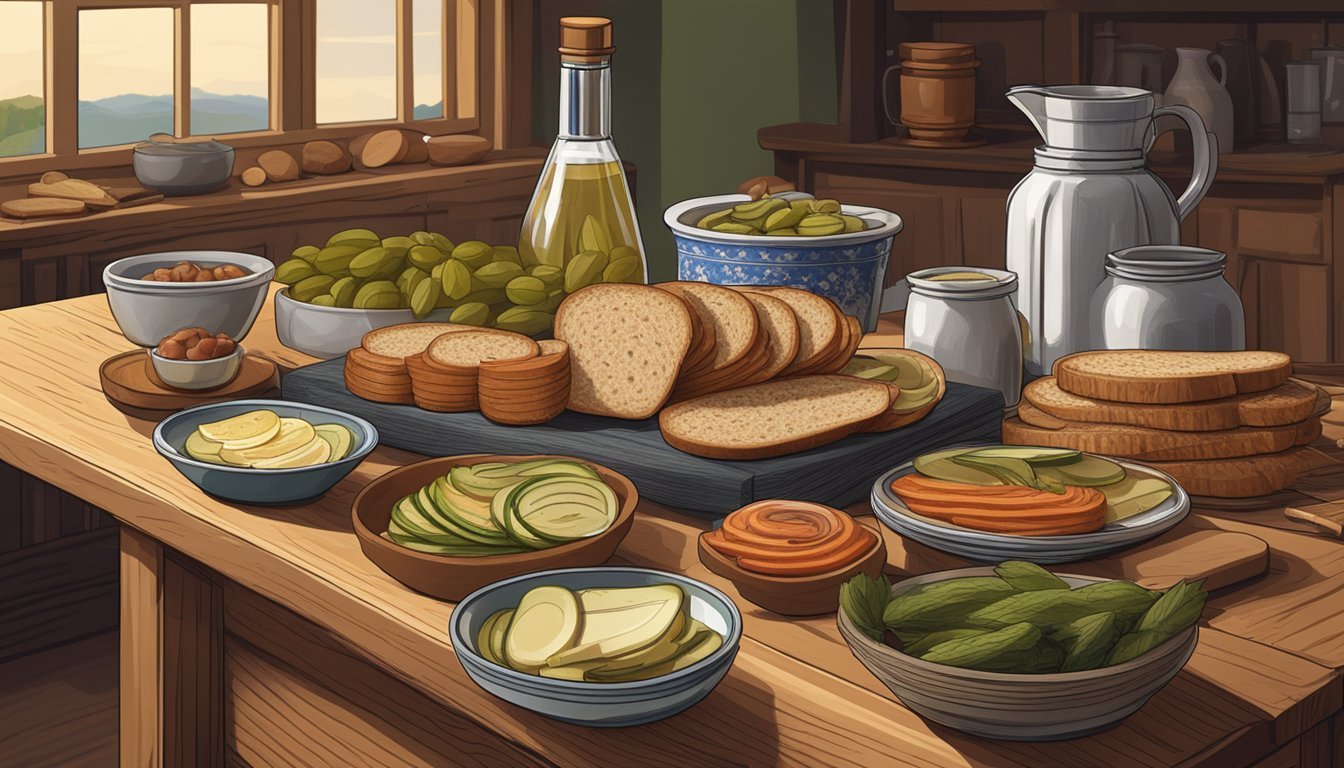The image showcases a detailed, animated cartoon-style illustration of a kitchen table laden with a variety of foods. At the forefront, there are multiple loaves of bread, avocados, lemon slices, and olives or almonds in an overflowing tin bowl. Carrot and corn husks are also scattered across the wooden table. On the right side of the table, there's a glass cruet containing olive oil and a metal jug with a yellow-green liquid, possibly pickle juice or another beverage, surrounded by metal or mason jar glasses. The scene includes bowls filled with assorted pickles, okra, cucumbers, and onion slices. In the background, a window reveals a daytime landscape with mountains in the distance, casting a natural light over the table. Cabinets filled with cups and containers are also visible on the right. The overall palette of the illustration is muted, with light browns, greens, and orangey-reds dominating the scene. This detailed, animated setting presents a cozy and abundant kitchen atmosphere.